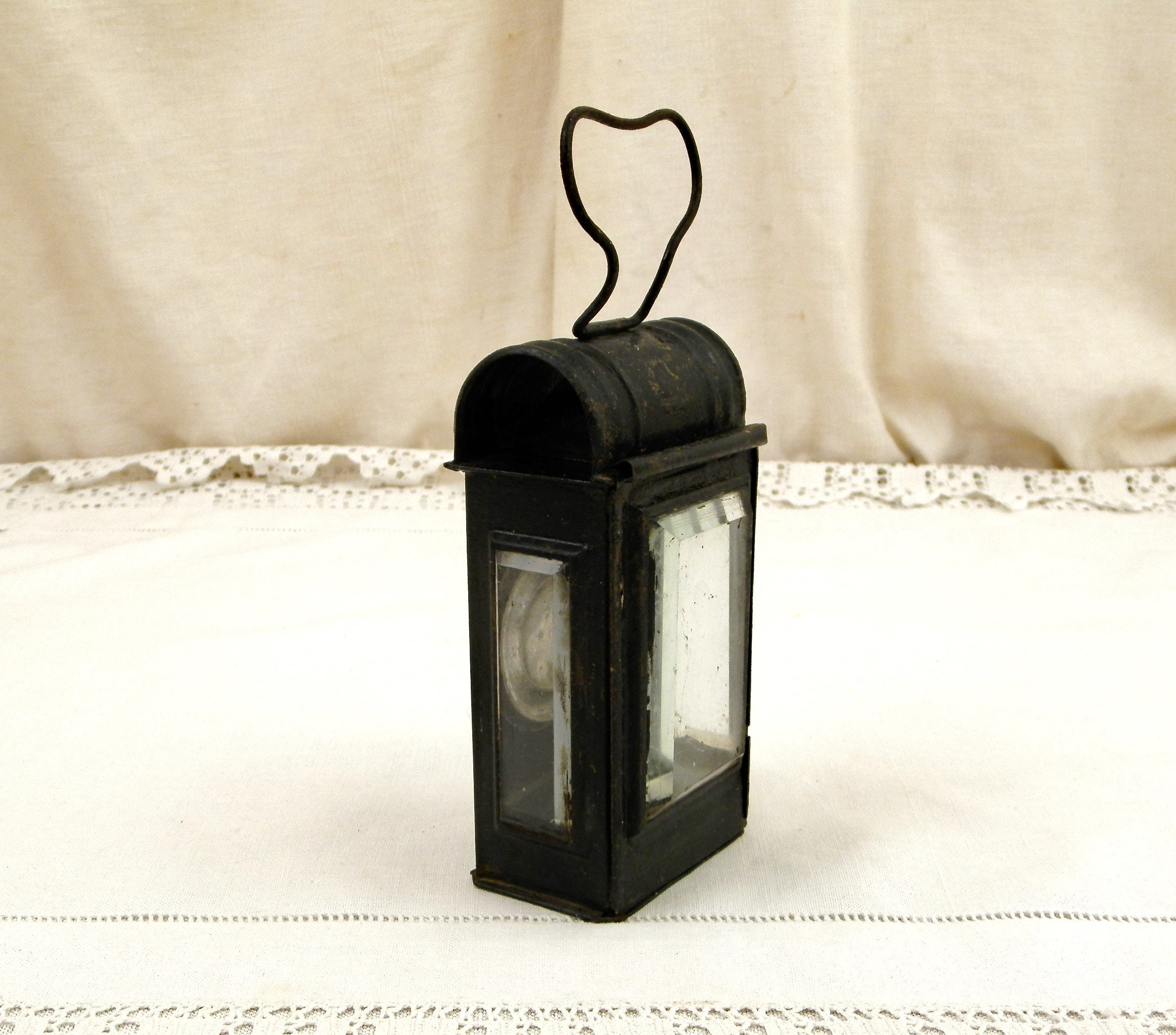This image depicts a vintage black metal lantern set against a lacy, off-white fabric background. The lantern, which appears to be an old-fashioned device, features a long, looped black wire handle and stands on an intricate lace-edged table runner. The lantern's top is rounded and resembles a half-barrel shape. Its design includes three vertical glass windows: a prominent one on the front and narrower windows on both the right and left sides. Through the window on the right side, a silver disc is visible. The image captures the lantern at an angle, showcasing its textured metal and plastic components, and is detailed with a cream to beige-hued fabric backdrop. This well-composed photograph could easily serve as an advertisement for an online marketplace, highlighting the antique charm of the lantern.